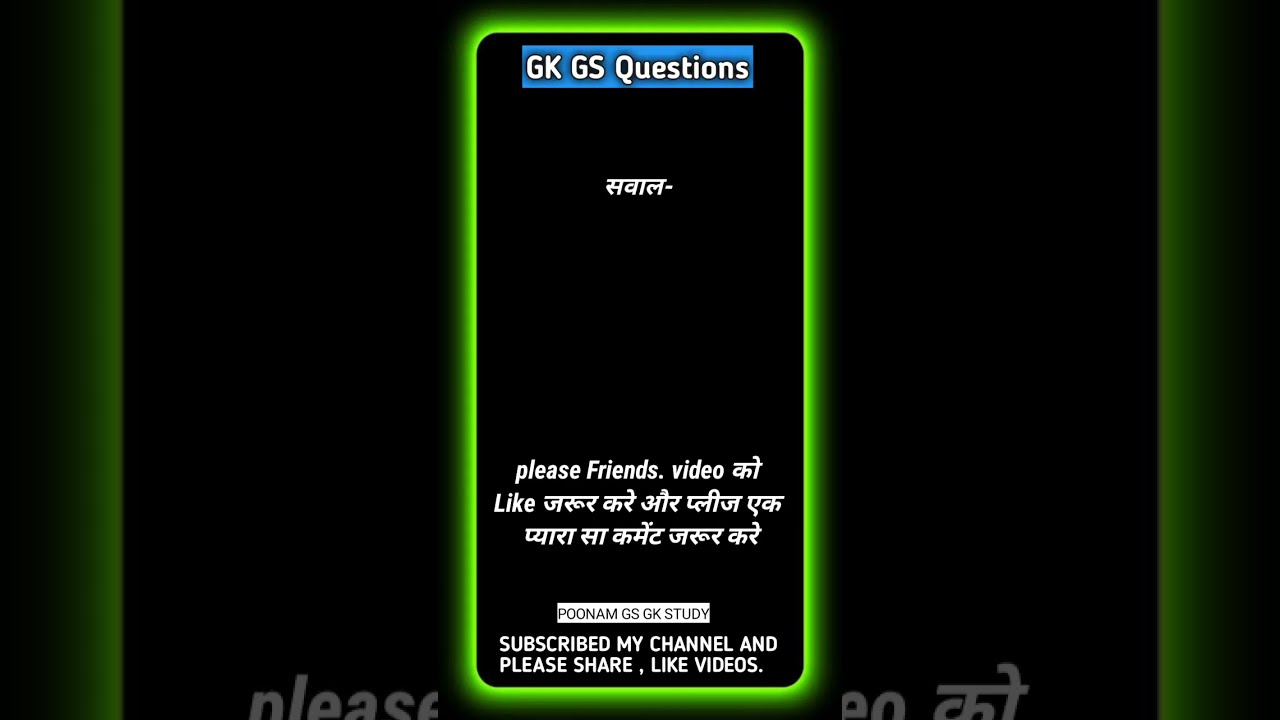The image is a detailed screenshot of a social media account, dominated by a distinctive green and black aesthetic. The backdrop features a neon green cell phone case with a black screen, centrally placed against the primary background. The account appears to integrate elements of video streaming or promotional content, indicated by the framing and layout.

At the top of the phone’s screen, a blue banner prominently displays the text "GKGS questions" in white font. Beneath this, several lines of text include a mix of English phrases and another language, possibly Middle Eastern, adding an international aspect to the content. The phrase "please friends video" is seen toward the lower part of the phone's display, followed by more non-English characters.

Further down, the text reads "Poonam GS GK study," with subsequent lines encouraging actions like subscribing, sharing, and liking videos. Specifically, at the very bottom, a message urges readers to "subscribe to my channel and please share like videos."

The entire image adheres to a horizontally rectangular format, enclosing the vertical, smartphone-shaped object. The visual style suggests it's a still shot from a video or a representation of a video streaming service page, emphasizing vivid colors such as neon green, blue, black, and white.